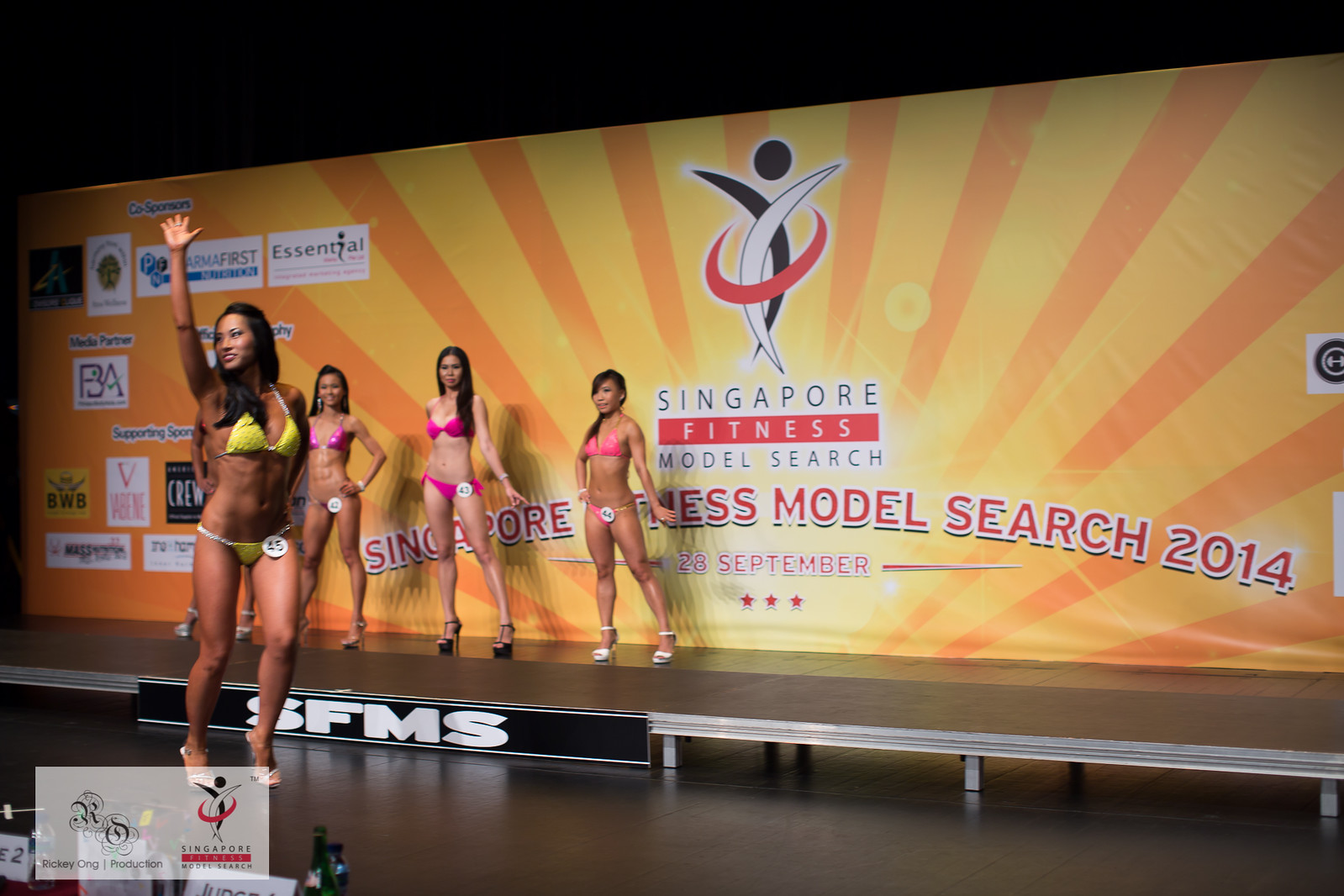This indoor photograph depicts a fitness model competition scene titled "Singapore Fitness Model Search 2014," held on September 28th. At the forefront, a model strides confidently from left to right wearing a yellow and white bikini, high heels, and the contestant number 45 pinned to her bikini bottoms. She is waving to the crowd with her right hand. Behind her, on a slightly elevated stage, stand four other models dressed in various shades of pink bikinis, each wearing high heels. The model furthest to the right sports a pink bikini with number 44, while next to her is a darker pink bikini-clad model numbered 43, and beside her is another model in a pink bikini with number 42. The fourth model, also in pink, is mostly obscured behind contestant 45.

The backdrop of the stage is vibrant with an orange and yellow striped design resembling sunbeams and contains multiple colorful logos on the left side. In the middle of this backdrop, large text reads "Singapore Fitness Model Search 2014, 28 September," accompanied by three stars below it. Additionally, a black bar with "SFMS" in white text is centered beneath the four women, and two black, white, and red logos are positioned in the lower corners of the image. This scene captures the essence and energy of the fitness competition, highlighting the participants' athleticism and the event's celebratory atmosphere.